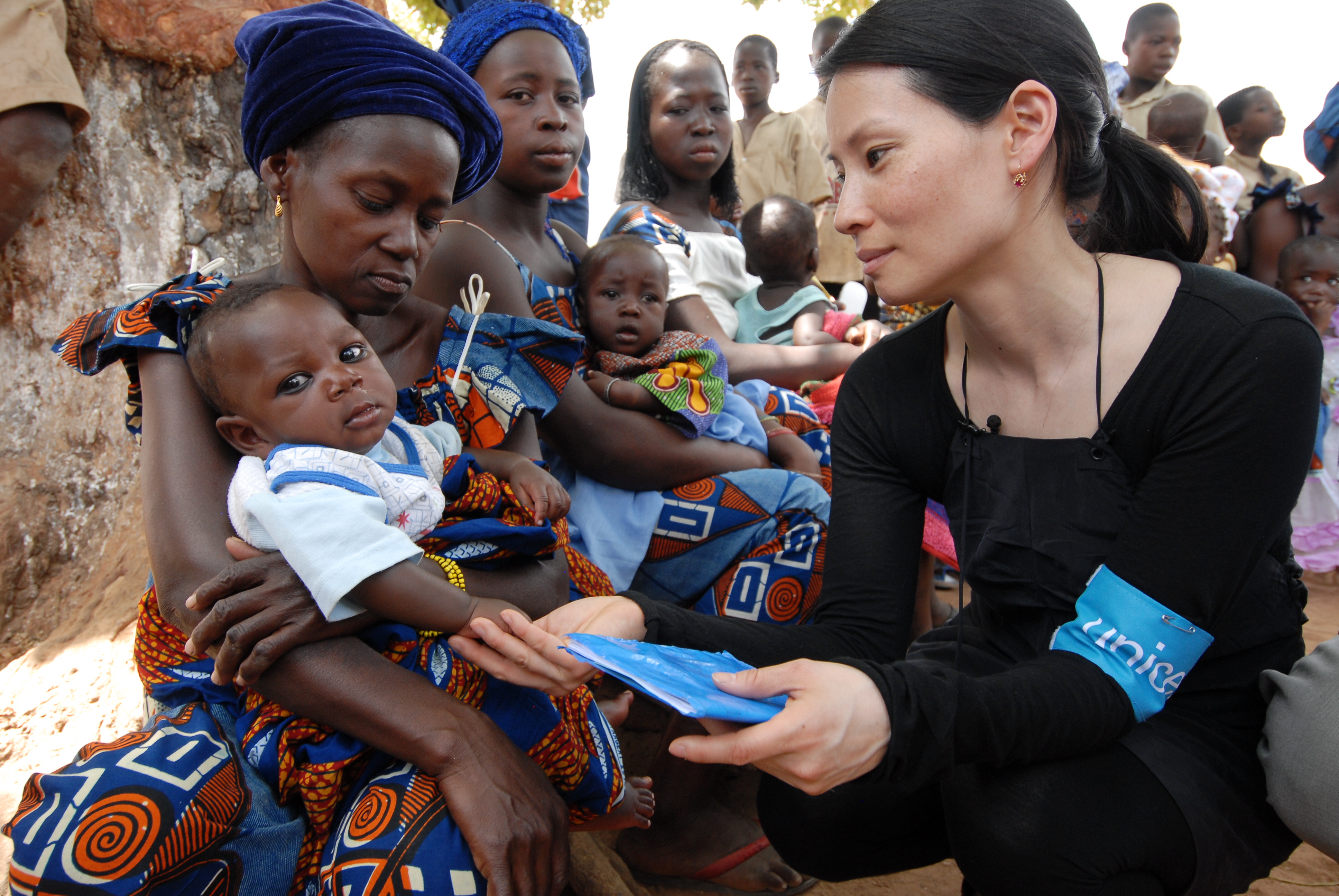In this photo, an Asian woman from UNICEF, dressed in an all-black outfit with a ponytail, is holding a blue plastic-covered pad and a booklet in her left hand. She is wearing a blue wrap around her left arm above the elbow. A large black leather strap hangs around her neck. The woman is gently touching the hand of a dark-skinned child, who is being held by his mother, a woman wearing a blue, orange, and white outfit and a purple turban. The mother is dressed in a robe with brown swirl designs and white patches, looking down at her child who is gazing sharply to the left. The scene is set outdoors, where a line of women with babies extends from the left side of the picture, curving out of view to the right. The gathering of mothers and their young children, possibly part of a UNICEF or UN program, seems to be seeking medical examination or assistance. No men are visible in the photo, only children, some of whom appear to be male teenagers. The overall atmosphere conveys a sense of anticipation and hope as the UNICEF worker assesses how to assist the community.